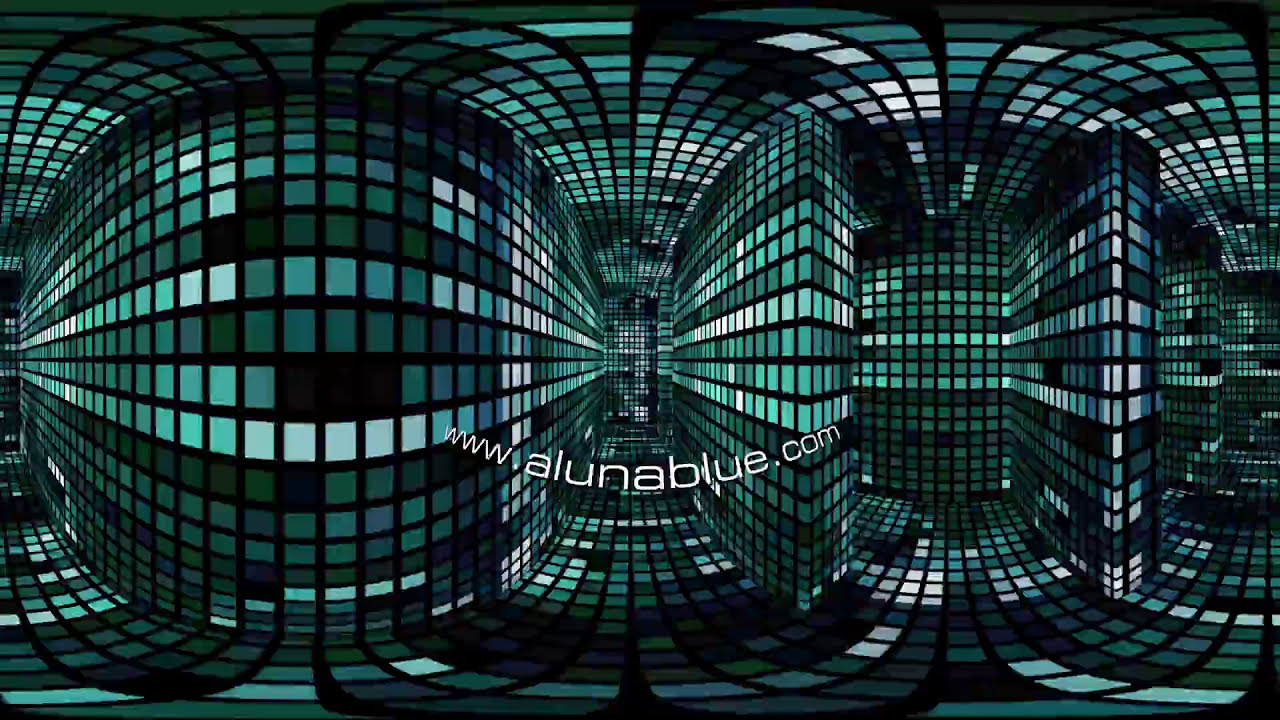The image showcases a surreal, kaleidoscopic hallway lined entirely with tiles in various shades of blue, green, grey, and white. The tiles cover the floor, walls, and ceiling, creating a mirror-like, 360-degree effect. The room appears endless, curving with no straight angles, and features several hallways extending in different directions, including one with a large black square on the left column. The scene is brightly lit, although there is no visible light source, as the tiles themselves seem to emit a glow. Overlaid on the image is the website address www.alunablue.com, written prominently in white font. The overall effect is mesmerizing, resembling a trippy kaleidoscope or an immersive digital art installation, with no people present in the hallway.